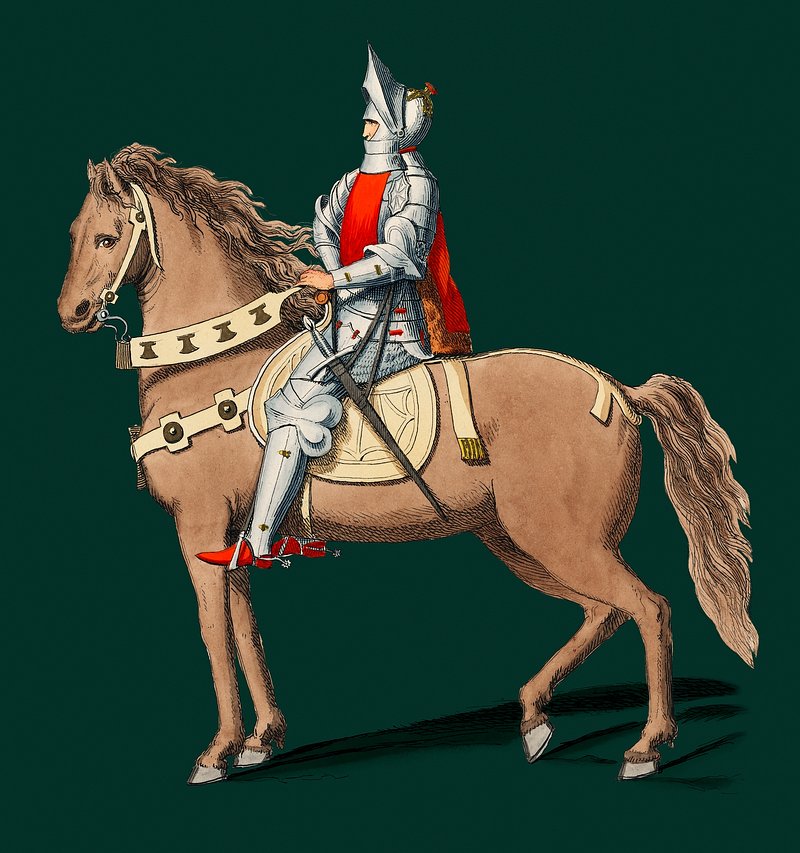This detailed illustration set against a solid dark green backdrop features a medieval knight riding a horse at the center of the image. The horse, facing toward the viewer, is a light brown or fawn color with a long, curly mane and tail, casting a shadow on the dark green background. The horse is adorned with a tan or pale yellow saddle and harness, both of which are decorated with axe-shaped markings and dark brown studs. Its gray hooves are clearly visible on the ground.

The knight atop the horse is clad in a full suit of silver armor, with only his eyes, nose, and part of his mouth visible through his upward-pointed open visor. He is wearing distinctive red shoes and a red cape that drapes down his back and across his chest. The top of his helmet features a golden crest with a red tip that matches the color of his cape. The intricate details of the knight's and horse's attire emphasize the historical and ornate nature of this vivid medieval scene.